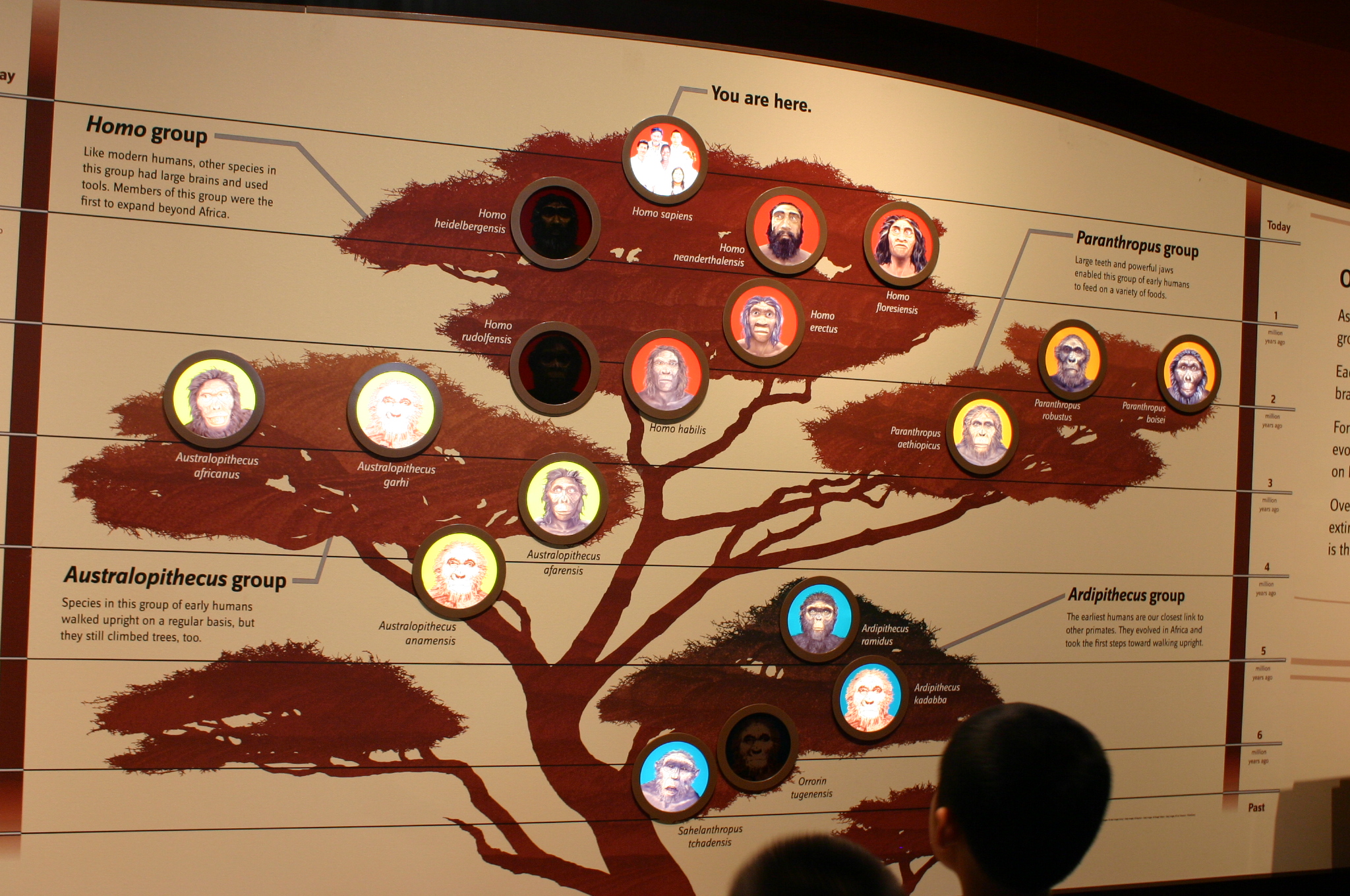This photograph captures a detailed wall mural depicting the evolutionary tree of humans, situated in a museum setting. Encased in a black frame against a deep red wall, the mural features a silhouette of a tree rendered in brownish-red hues on an off-white backdrop. The branches of the tree illustrate various stages of human evolution, each with accompanying images of different hominin faces.

At the very top of the tree, the text "You are here" marks the location of modern humans, Homo sapiens. To the left of this, the "Homo group" is highlighted with the note that species within this group had large brains, used tools, and were the first to expand beyond Africa. Descending further, the "Paranthropus group" is situated to the right, though the smaller descriptive text is less legible. On the lower left, the "Australopithecus group" is identified, indicating that these early humans walked upright regularly but still climbed trees. Positioned at the lowest point of the tree on the right, the "Ardipithecus group" is noted, with text that is nearly impossible to read. The mural clearly delineates these four primary evolutionary groups, offering a visually comprehensive guide to human evolution.